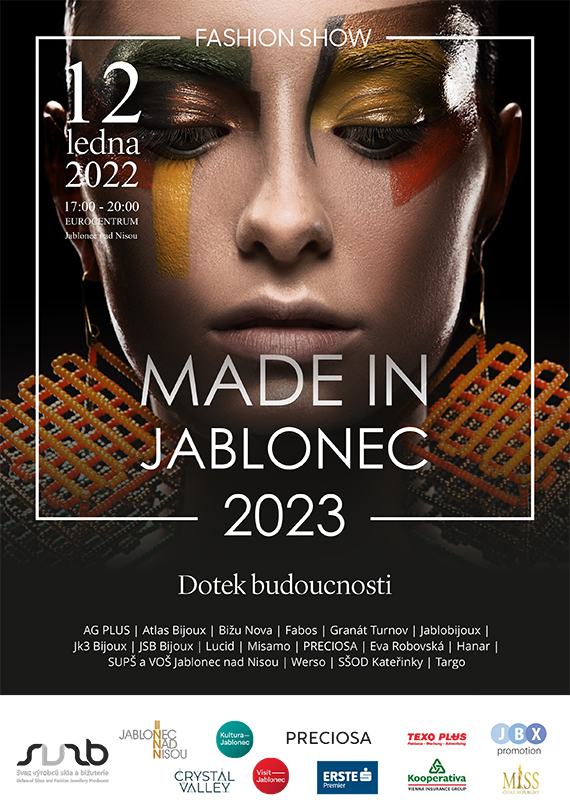The image is a detailed color photograph in portrait orientation, serving as a promotional piece for a fashion show. Dominating the background is a close-up of a woman's face, from mid-forehead to the middle of her neck. She gazes downward, her face adorned with bold, asymmetrical geometric makeup in shades of bronze, red, and gold. She has a bronze complexion and wears large triangular earrings made from a gridwork of orange plastic material. Surrounding the central image is a thin white rule. At the top, in white text, it reads "Fashion Show." Below this, on the left, is the date "12 Ledna 2020, 1700 to 2000," and the prominent text "Made in Jablonek, 2023." Below this, several sponsors’ names and logos are listed, including SURB, Preciosa, Texo Plus, S3, Crystal Valley, and JBX. The background behind the model is black, making the white text stand out prominently. The overall style merges photographic realism with graphic design elements.